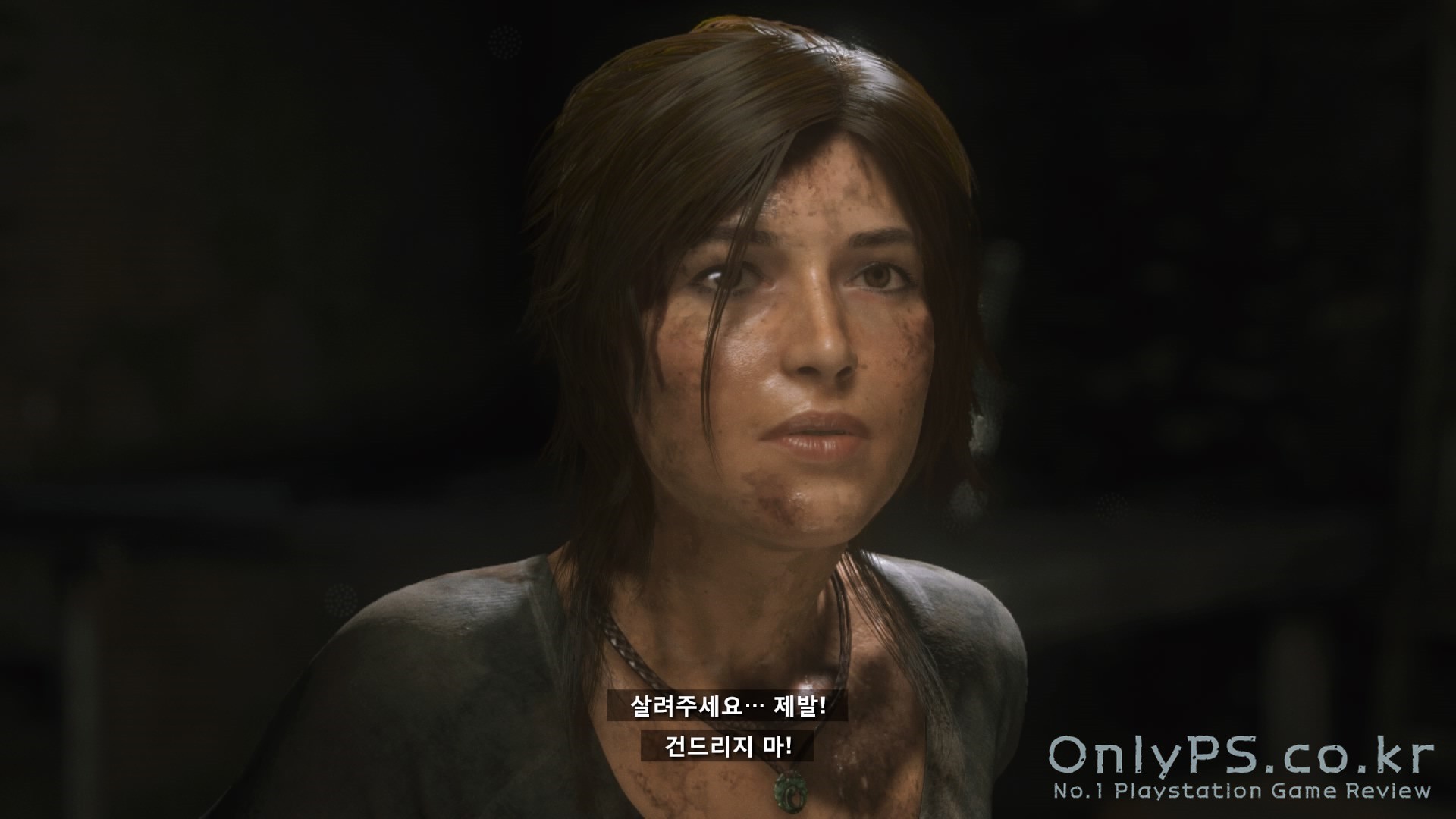This image appears to be a screenshot from a video game, featuring a female character prominently at the center. The woman has short, dark hair parted in the middle, with a noticeable strand hanging over her right eye and falling around the top of her chest, just where the neck begins. Her face and clothes are heavily soiled with dirt and grime, enhancing the rugged and gritty atmosphere of the scene. She is dressed in a low-cut gray shirt and wears a metal necklace. The background behind her is dark, with a table faintly visible, adding to the ominous and mysterious setting. At the bottom center of the screenshot, subtitles in white Asian characters can be seen, though their specific language remains unclear. In the bottom right corner, the text "onlyps.co.kr Number one PlayStation Game Review" is displayed in white font, indicating the source's evaluation of the game.